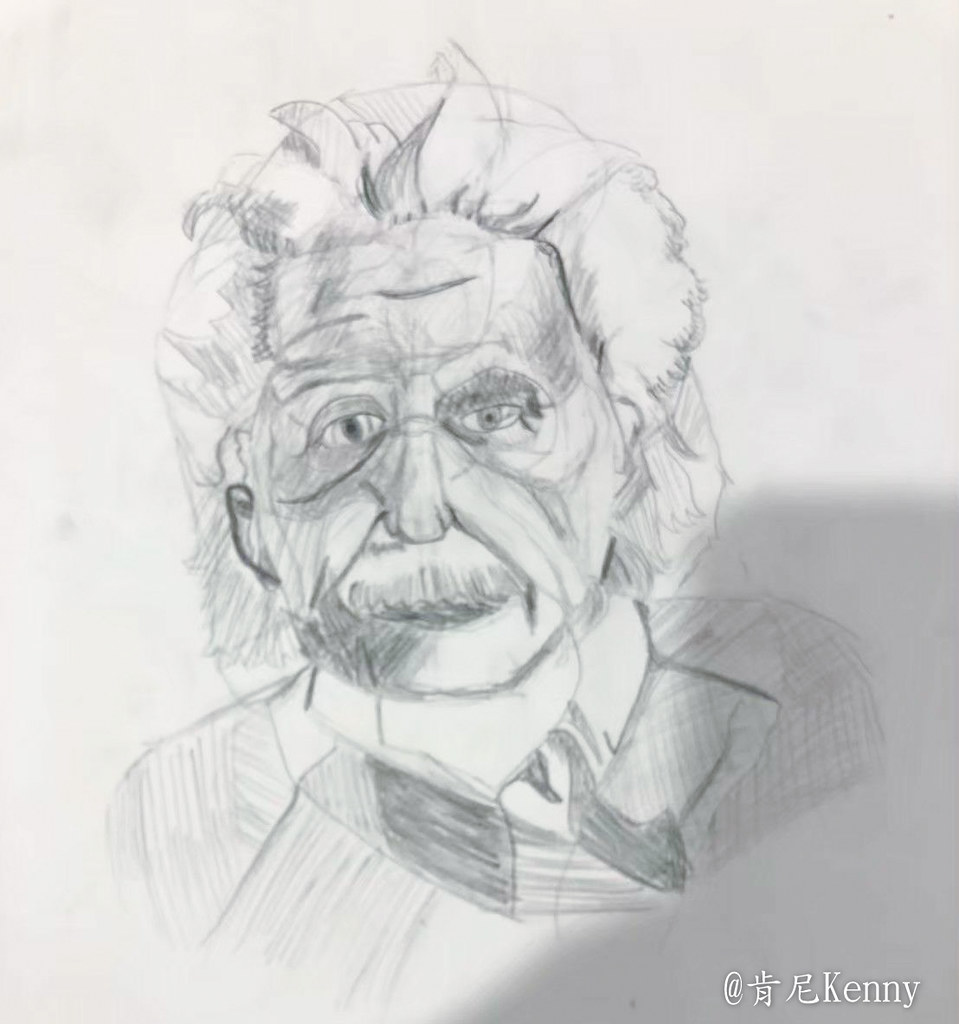This detailed pencil sketch captures the iconic image of an elderly Albert Einstein. The lifelike depiction showcases Einstein with his characteristic thick, full mustache and a head of wild, white hair. He is portrayed wearing a collar and an untied bow tie, lending an air of casual intellect to the distinguished physicist. Einstein’s gaze is directed straight at the viewer, creating an engaging and direct connection. The portrait is in a vertical orientation, set against a slight off-white or light gray background that accentuates the intricacy of the sketch. In the bottom right corner of the artwork, credits are given in a foreign script along with the name "Kenny," indicating the artist.